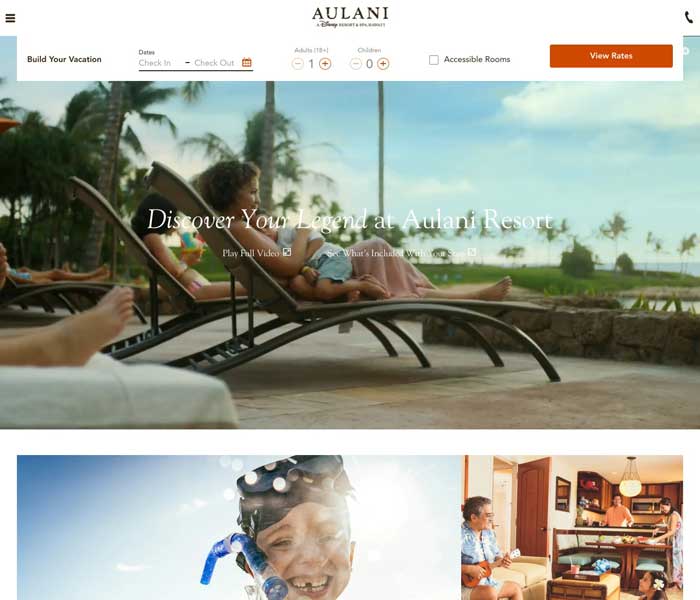**Descriptive Caption:**

The webpage for Alani, a Disney Resort, features a vibrant and inviting layout that highlights the luxurious and family-friendly atmosphere of the resort. The centerpiece of the page is a captivating image of a beachside scene. In the foreground, a joyful black woman reclines on a beach chair with her child resting comfortably on her lap. The serene setting is complemented by palm trees and crystal-clear water in the background, evoking a sense of paradise. Behind them, another woman enjoys a refreshing drink, adding to the relaxed, holiday vibe.

Below this, there is an endearing photograph of a young child smiling brightly, missing both sets of his front teeth. He wears a pair of goggles and has a blue snorkel hanging off the side of his face, with the sun casting a warm glow behind him, highlighting his playful and adventurous spirit.

Further down, an image captures a warm family moment inside what appears to be a cozy lodging area. An elderly man serenades those around him with a ukulele from the couch. Nearby, one person sets the table while another is busy in the background kitchen, and a child looks up admiringly at the musician. The scene is made homier by the presence of a drink and a board game placed on a small ottoman in front of them.

At the top left of the page, a context menu helps users customize their vacation plans, including options to select dates for check-in and check-out, the number of adults and children, and the choice for accessible rooms. An orange 'View Rates' button below the menu facilitates easy navigation. The top right hand side prominently features a call button for immediate assistance.

The page is visually unified with the slogan "Discover Your Legend at Alani Resorts" displayed in elegant white lettering over the main image, emphasizing the enchanting and legendary experiences awaiting visitors at Alani, a Disney Resort.